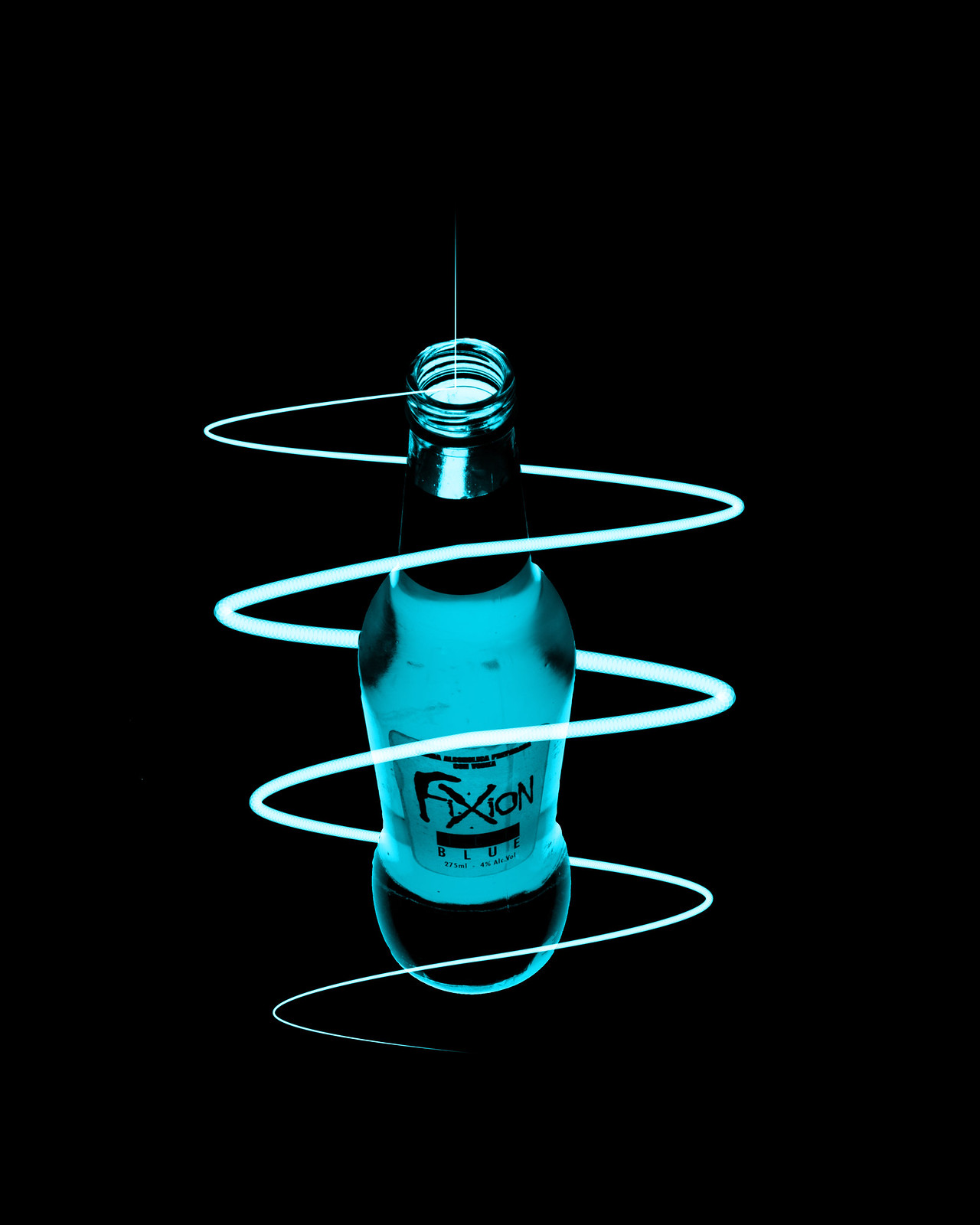Displayed against an entirely black background, the image features a blue bottle that appears to be part of an advertisement for a beverage called "FIXION Blue." The label on the bottle spells out "FIXION" in capital black letters, with a black rectangle beneath it indicating the word "Blue," along with details on the milliliter content and alcohol percentage. A distinctive neon blue corkscrew-like light spiral starts at the mouth of the bottle, encasing it in a futuristic glow that adds a dynamic visual effect. The bottle displays a contrast of black and blue hues: the mouthpiece and bottom are black, while the main body is illuminated in a striking blue tone. The photo captures the vibrant, squiggly laser-like light that wraps around the bottle, emphasizing the modern and sleek design of the product. This minimalistic yet eye-catching composition strongly suggests that the image is an advertisement, creating an aura of mystery and sophistication around the bottled product.